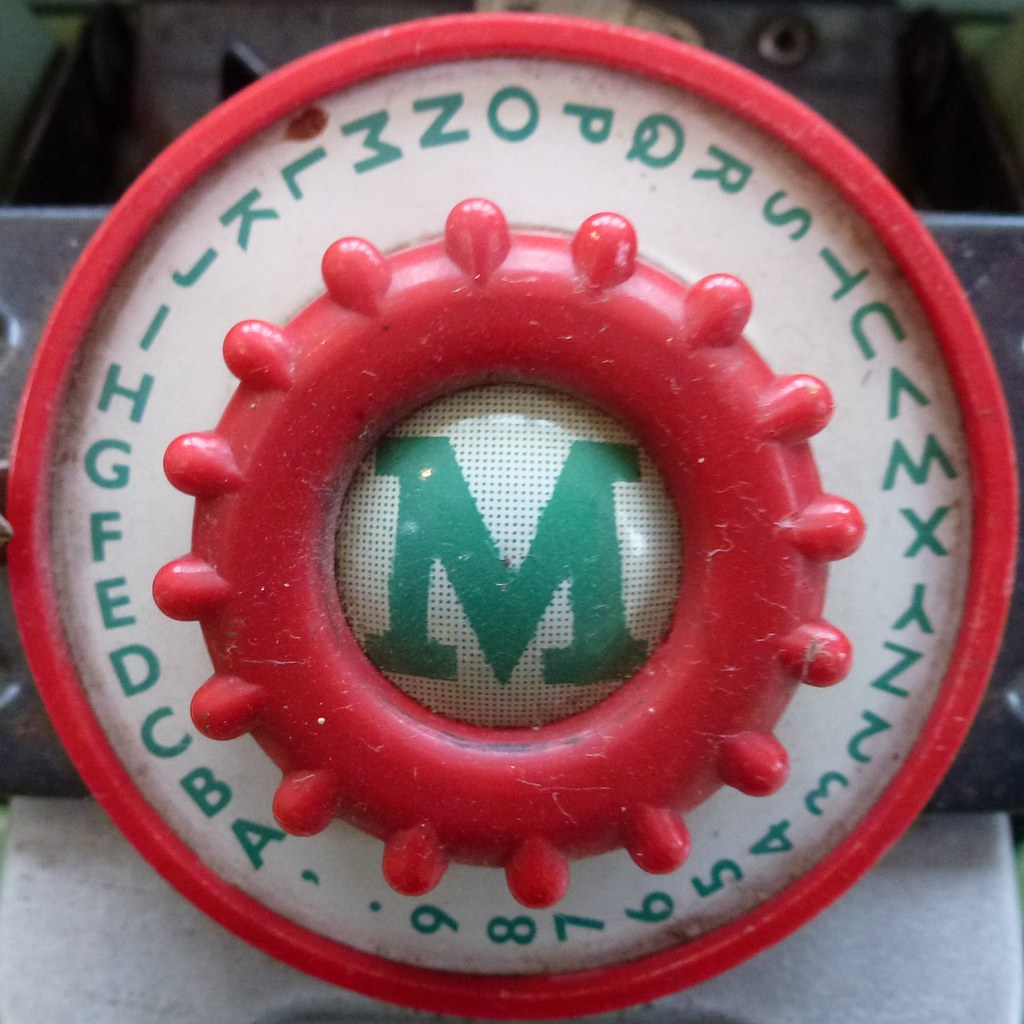The image features a circular child's toy, likely designed for educational purposes. The toy is primarily made of red plastic forming its outer border. Inside this border is a white background adorned with green letters of the alphabet and numbers. At the center of the toy lies a green "M" enclosed within a smaller circle. Surrounding the "M" are multiple dots. The toy includes a dial mechanism that suggests it can be turned to select different numbers or letters. The image appears to show the toy resting on a table, although the background details are indistinct.